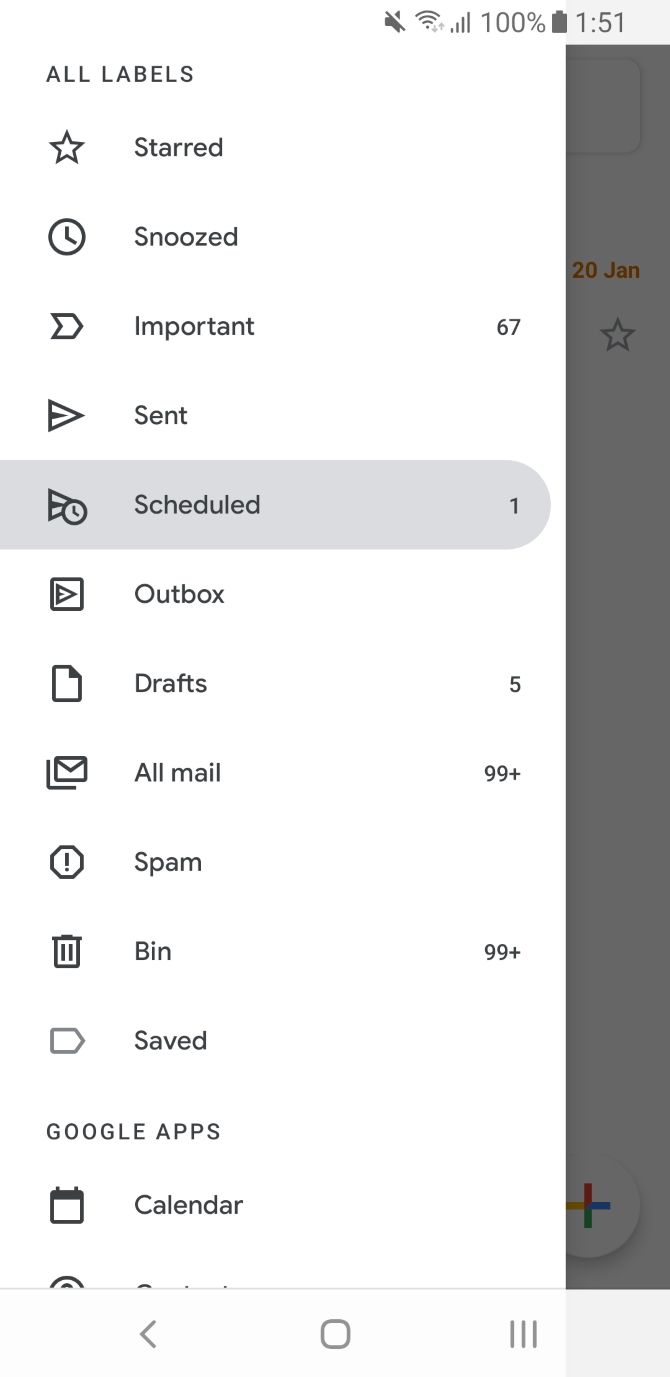The image depicts a user interface that appears to be from a mobile email application. 

In the top right corner, there are several status icons: first a muted sound symbol, followed by a WiFi symbol. Next to these, four signal bars get progressively taller from left to right, indicating full signal strength. Adjacent to this, there's a fully charged battery icon displaying "100%." Just below these icons, a section with a gray background displays "1:51."

On the top left-hand side, the label "All labels" can be seen. Below this, there are several icons each followed by descriptive text: 
- A star icon labeled "Starred"
- A clock icon labeled "Snoozed"
- An arrow icon labeled "Important"
- A triangle with a line through it labeled "Sent"

Further down, a gray rectangular button with a bulging right side features a triangle with a clock on it labeled "Scheduled." Next, a square with a triangle inside is labeled "Outbox," and a sheet of paper with a folded corner is labeled "Drafts." An envelope icon with a line to the left is labeled "All Mail," a geometric shape with an exclamation point inside is labeled "Spam," and a trash can icon is labeled "Bin."

Additional icons include:
- An arrow pointing right labeled "Saved"
- A Google app icon
- A calendar icon labeled "Calendar"

The bottom of the Calendar label is partially obscured.

On the right side of the screen, there's a vertical gray bar with numbers displayed intermittently. About one quarter down this bar, an orange label with "20 JAN" and a gray-outlined star is visible. A partially visible white and light gray circle with a multicolored plus sign is also present.

Finally, at the very bottom of the interface are three icons: a left-pointing arrow, a square, and three horizontal lines, ending with a light gray box.